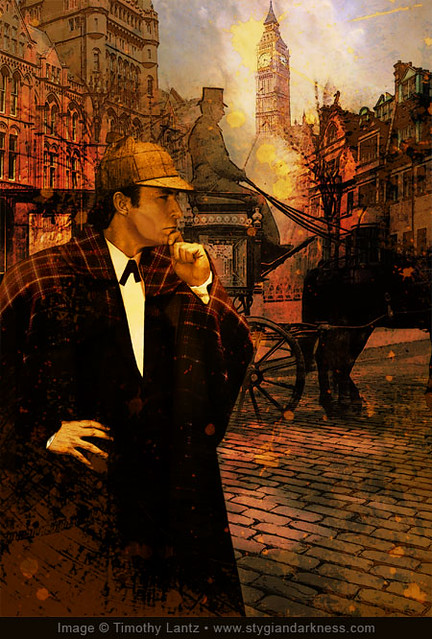The detailed artwork by Timothy Lance, prominently featuring the website www.stygiananddarkness.com at the bottom, depicts a scene reminiscent of Sherlock Holmes' era. At the forefront stands a white male dressed in a sophisticated ensemble: a white collared shirt beneath a black coat, topped with a plaid jacket in shades of yellow, red, and brown. His matching plaid hat, with a brim, completes the Sherlock Holmes look. Striking a pensive pose, he rests his hand on his chin and gazes thoughtfully to the left. Behind him unfolds a dramatic backdrop of a city in turmoil, with towering buildings seemingly engulfed in flames. Notably, a horse-drawn carriage with a black horse is discernible on the right, showcasing the driver atop a high buggy seat. The cobblestone streets add to the old-world charm and depth of the vibrant, yet chaotic, watercolor-like scene, accentuated by splotches of yellow and red.